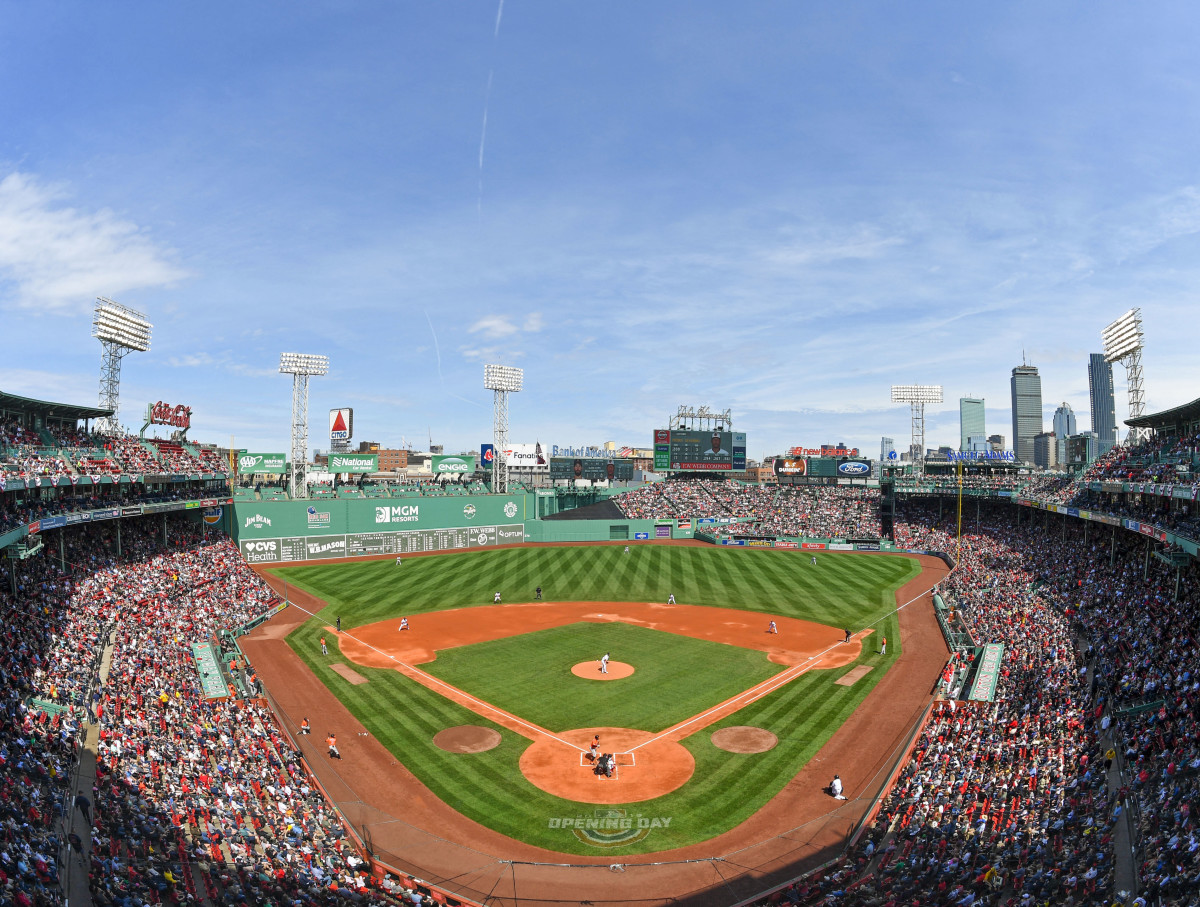This image captures an exhilarating moment during a baseball game on opening day, viewed from a high vantage point, likely an upper stand. The top half of the photo reveals a clear blue sky streaked with white, feathery clouds, setting a picturesque backdrop for the event. The green field below is meticulously maintained with rich, darker green vertical stripes. Tiny players are visible on the field, occupying their traditional positions.

The stadium is buzzing with energy, evidenced by packed stands with no empty seats. Five spotlights are strategically placed around the stadium, and various advertisement signs, including Citgo, Coca-Cola, and Ford, are visible in the background. The perspective offers a semi-bird's eye view, giving a comprehensive look at the stadium's vibrant atmosphere on a sunny day.